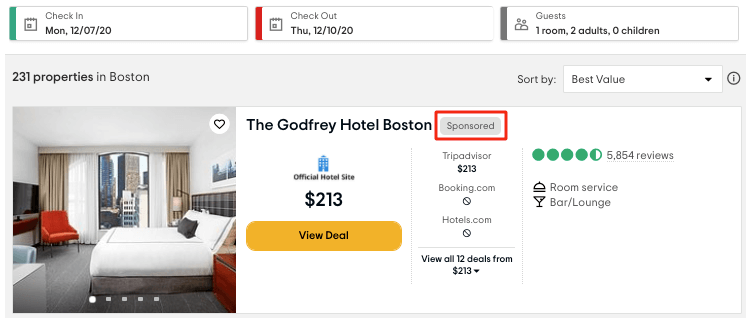**Caption:**

The Godfrey Hotel Boston, available for $213 per night, offers a prime location in downtown Boston with amenities illustrated in this screenshot. The booking, made on a travel discount site, details a three-day stay from December 7 to December 10, 2020, for one room accommodating two adults. This upscale hotel boasts a modern, bright room with a flat-screen TV, comfortable bedding, and an outstanding view of the city. The Godfrey holds a high rating of 4.5 stars based on nearly 6,000 reviews. As noted, only TripAdvisor is offering this deal, highlighting its exclusivity on this particular platform.